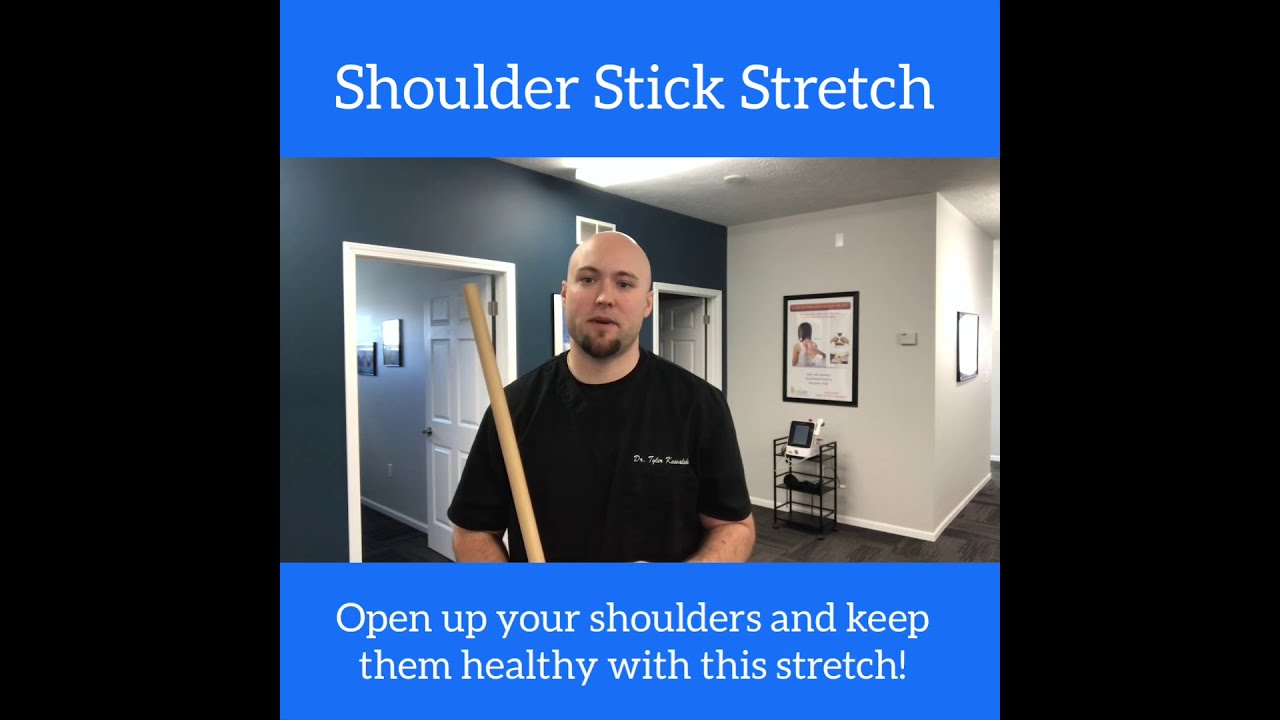In a photograph titled "Shoulder Stick Stretch," text in white font on blue rectangular banners appears above and below the central image. The upper text reads, "Shoulder Stick Stretch," while the lower text instructs, "Open up your shoulders and keep them healthy with this stretch." The man in the center of the photograph, presumably named Dr. Tyler Ramirez as indicated by the text on his short-sleeved black t-shirt, is bald and has a brown goatee. He is in an office-like room characterized by white walls and ceilings, with a teal or dark blue accent wall featuring two white doors and what appears to be medical posters. The man holds a stick, likely to demonstrate the shoulder stretch described in the text. Additional details in the background include a black bookshelf and brown tiled flooring, suggesting a space designed for physical therapy or medical recovery exercises. The edges of the entire image are bordered by black rectangles, adding a frame-like effect to the composition. The setting, complete with medical or instructional posters, hints that this image might be a screen capture from an instructional or recovery video.